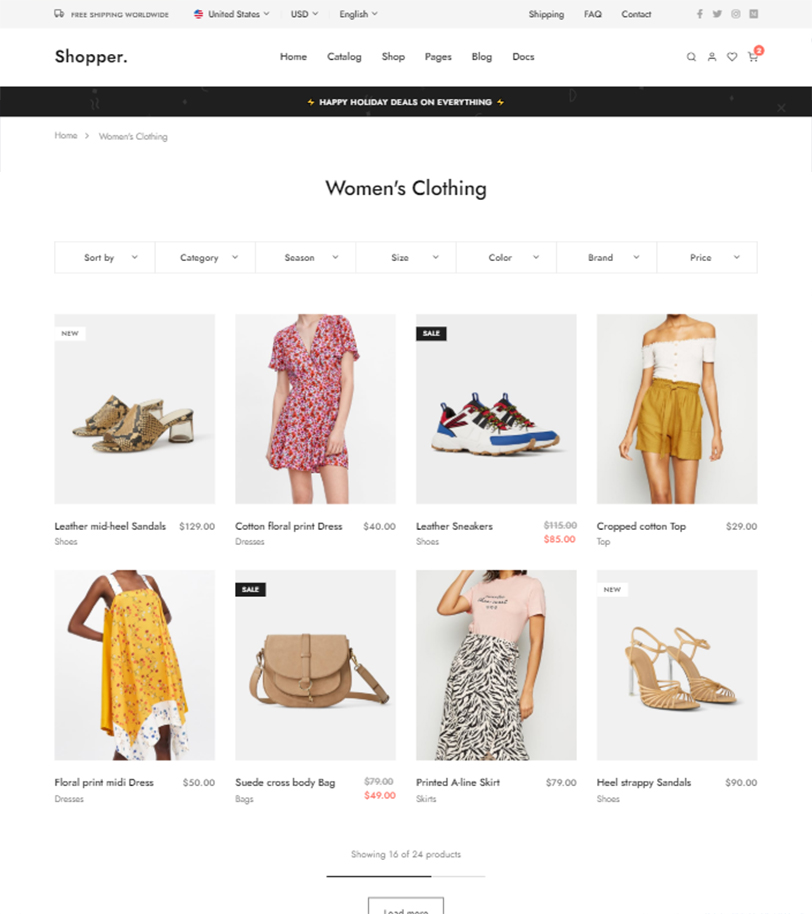This screenshot showcases the home page of a website named "Shopper," prominently featuring its navigation bar at the top which includes various categories such as Home, Catalog, Shop, Pages, Blog, and Docs. Accompanying these are standard website icons like a search bar, a user profile icon, a heart for favorites, and a cart icon. Below this navigation bar is a black banner displaying "Happy Holiday Deals on Everything."

The primary section of the page indicates that the viewer is on the "Women's Clothing" section under the Home category. This section provides options to filter products by various criteria such as Sort By, Category, Season, Size, Color, Brand, and Price, each equipped with a dropdown arrow for further customization.

Displayed in the main content area are images of eight different fashion items:
1. Leather mid-heel sandals in tan brown priced at $129.
2. A cotton floral print dress featuring pink, red, and blue colors for $40.
3. Leather sneakers in red, white, blue, and black originally priced at $115, now on sale for $85.
4. A white cropped cotton top paired with mustard yellow shorts for $29.
5. A floral print midi dress in white and yellow polka dots for $50.
6. A suede crossbody bag priced at $79, now discounted to $49, available in tan.
7. A printed A-line skirt in black and white resembling a leopard or zebra pattern, modeled with a pink t-shirt.
8. Tan heel strappy sandals priced at $90.

Each item is visually represented, providing a detailed overview for shoppers browsing through women's clothing.